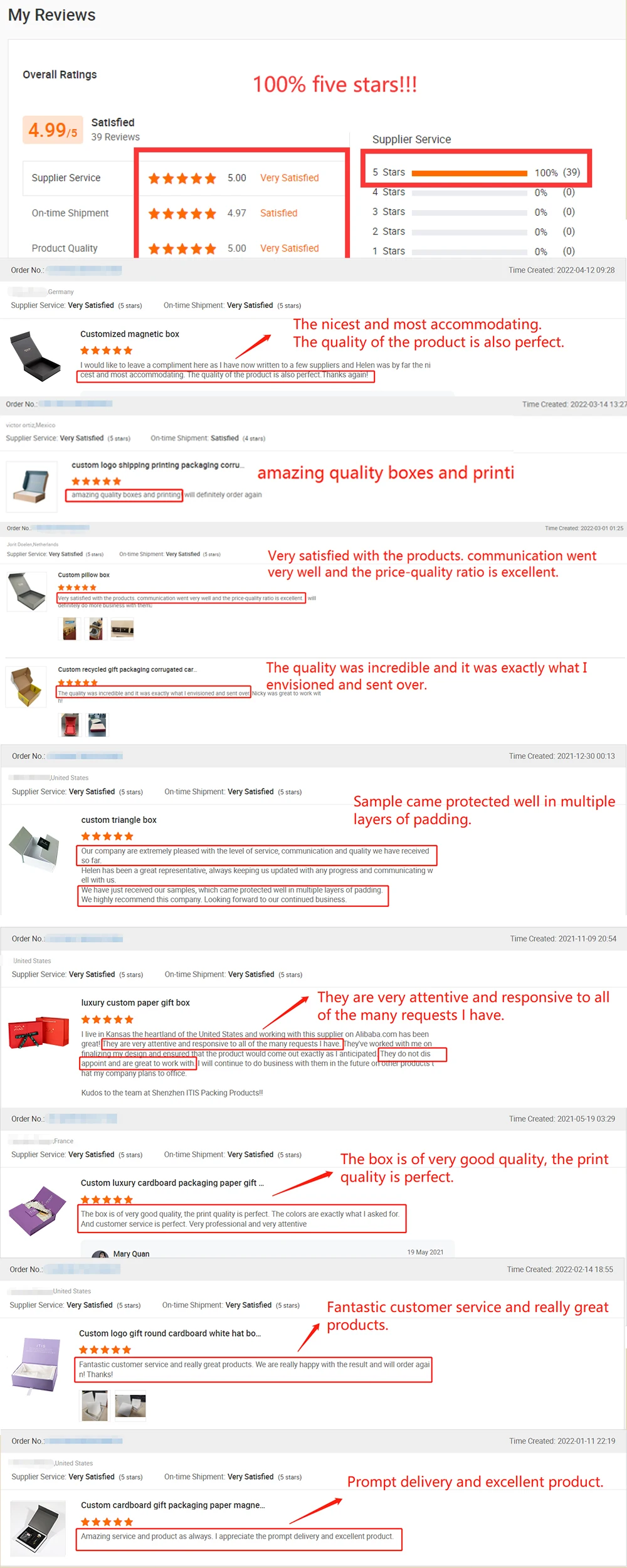**Detailed Caption:**

This image is a screenshot from a device, showcasing a detailed review section on a webpage. At the top of the screenshot, the heading "My Reviews" is prominently displayed in grey text. Below this, within a white rectangular section, it reads "Overall Ratings," and the rating is featured as 4.99 out of 5 within a faded orange rectangle, which contains orange text. Beneath this, the word "Satisfied" is highlighted in bold black text, followed by the note, "39 reviews," in grey.

In the center of the image, the text "100% 5 stars" stands out in red. On the left-hand side, various aspects of the rating are listed in black text, including "Supplier Service," "On-Time Shipment," and "Product Quality." Each of these categories is accompanied by an overall star rating, with "Supplier Service" and "Product Quality" both receiving 5 out of 5 stars. "On-Time Shipment" has a slightly lower rating of 4.97, but still displays mostly full orange stars.

Additionally, a section labeled "Supplier Service" shows an impressive 5-star rating with 100% satisfaction from 39 reviewers. The image also depicts several purchased items cascading down the page, although the text describing these items is too small to read clearly. This screenshot captures a comprehensive and highly positive review overview for a supplier's services and products.